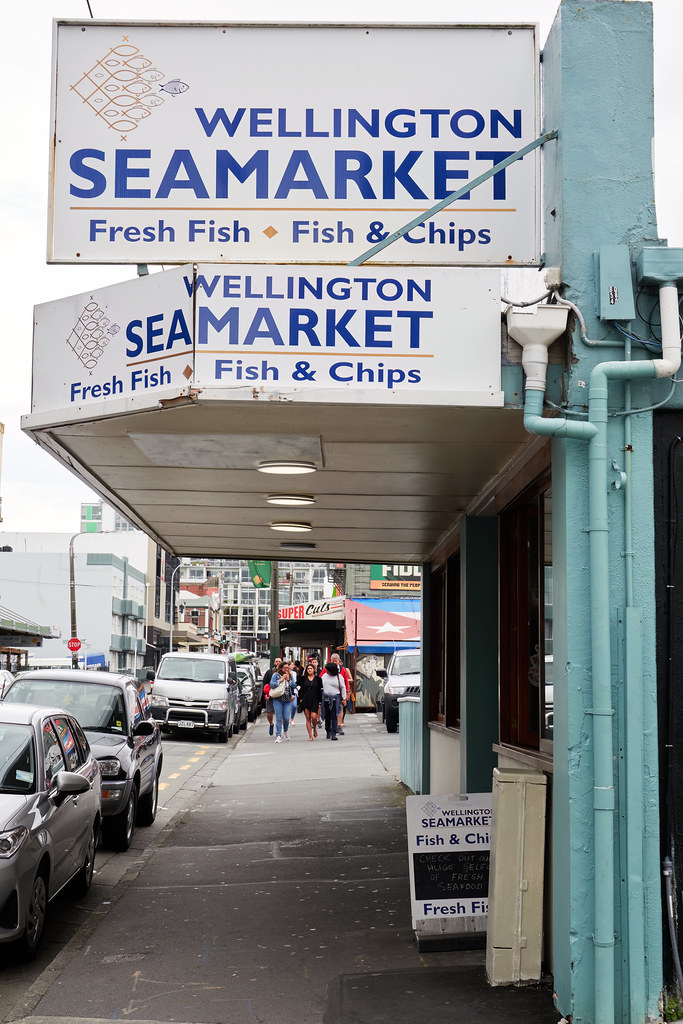In this photograph taken from the perspective of a sidewalk on a cloudy day, the immediate foreground features a storefront with a teal side and a white marquee adorned with blue lettering that reads "Wellington Sea Market Fresh Fish, Fish and Chips." The awning and a larger sign above also repeat this name and menu. Small lights are visible under the marquee, adding a gentle illumination. Several cars are parked along the edge of the sidewalk. In the distance, a substantial group of people walk towards the camera, contributing to a bustling city sidewalk atmosphere. Additional signage, possibly a billboard, is present on the lower right side. The building housing the store is painted blue, with visible pipes contributing to the urban setting's character.